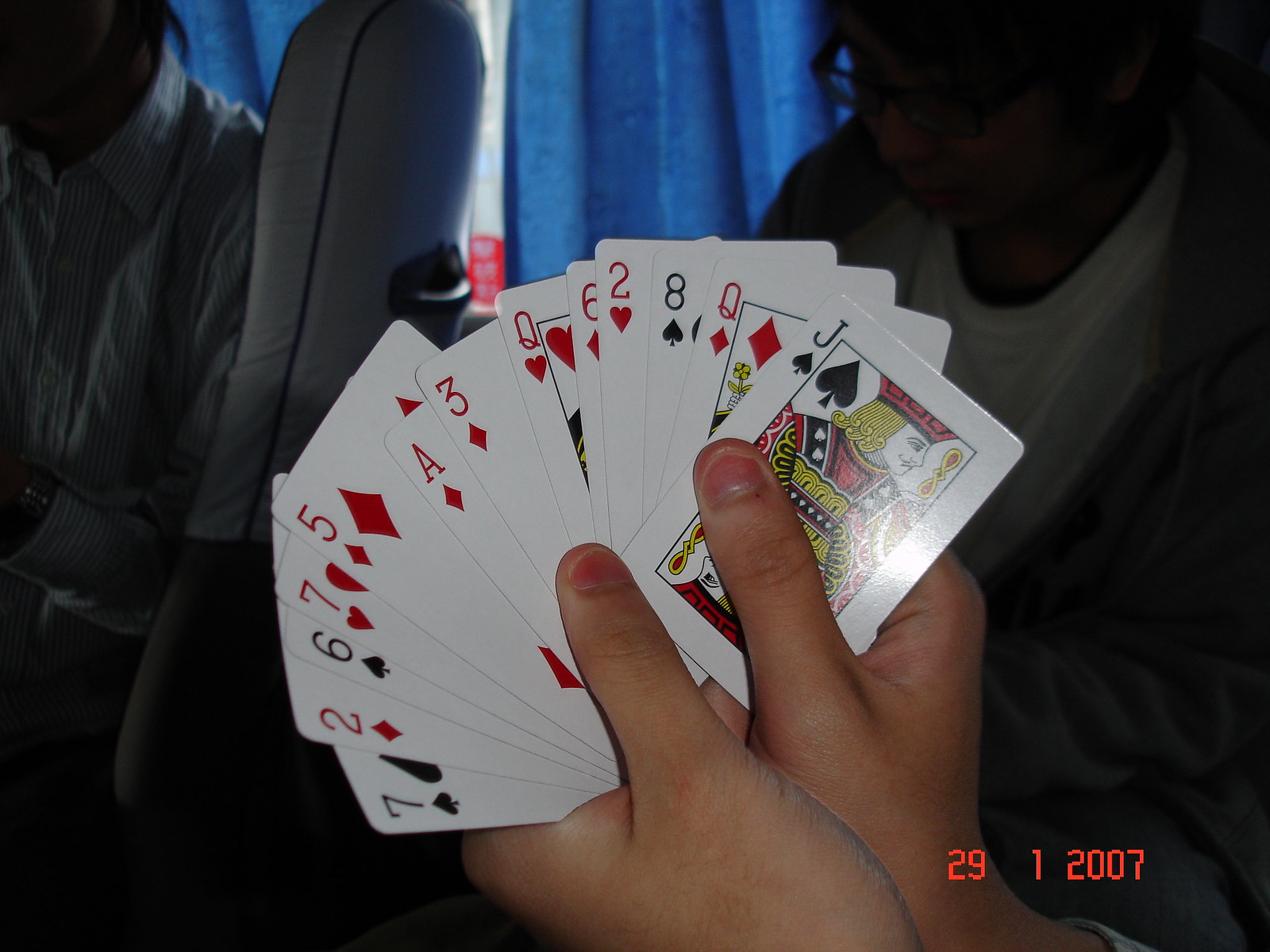In the image, two closely-cropped, white hands are holding a fan of 14 playing cards. These cards, splayed out for visibility, include the 7 of Spades, 2 of Diamonds, 6 of Spades, 7 of Hearts, 5 of Diamonds, 8 of Diamonds, 3 of Diamonds, Queen of Hearts, 6 of Diamonds, 2 of Hearts, 8 of Spades, Queen of Diamonds, and a Jack of Spades. The timestamp on the bottom right corner indicates the date as January 29th, 2007. The gender of the individual holding the cards is ambiguous, as no definitive traits can be determined. The fingers are neatly trimmed, and part of a sleeve is visible on the wrist.

The background of the image is dark, making it difficult to discern details. There appears to be the silhouette of another person adjacent to the cardholder, though their face remains obscured. This person has some hair visible behind what looks like a pair of glasses. A faint white object can be seen in the foreground, but it is indiscernibly blurry.

To the left side of the image, there is likely another person dressed in dark clothing, but their features are also unclear. In the background, a window with blue curtains partially visible adds a subtle hint of light, but does not significantly illuminate the scene. The primary focus remains on the two hands gracefully displaying the array of playing cards.